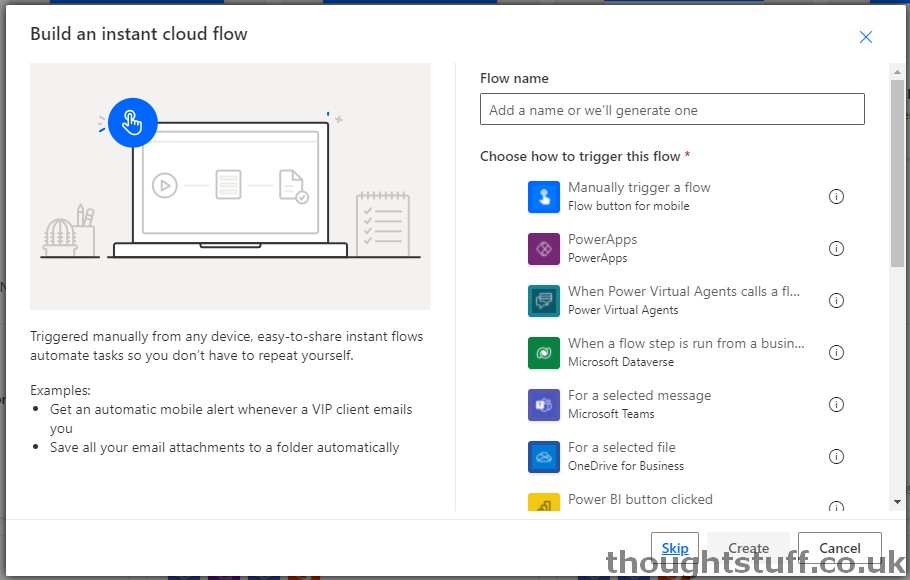The image displays a screenshot of a website hosted at ThoughtStuff.co.uk, as indicated in the bottom-right corner. Central to the image is a black-outlined white box. At the top inside this box, the text "Build an Instant Cloud Flow" is prominently displayed in black. Below this heading, there is a grey rectangle featuring an illustration of a desk. The desk includes an open laptop, a pencil holder, a small cactus plant on the left, and a notebook situated to the right of the laptop. Additionally, there is a blue clicking icon located at the top-left of the page.

Beneath the desk illustration, there is space dedicated to text and key points, offering examples relevant to the topic. To the right of these examples, there is a field labeled "Full Name" accompanied by a box with the instruction to "Add a name or we will generate one." Further down, a section is titled "Choose how to trigger this flow," which presents multiple options with corresponding informational buttons to the right.